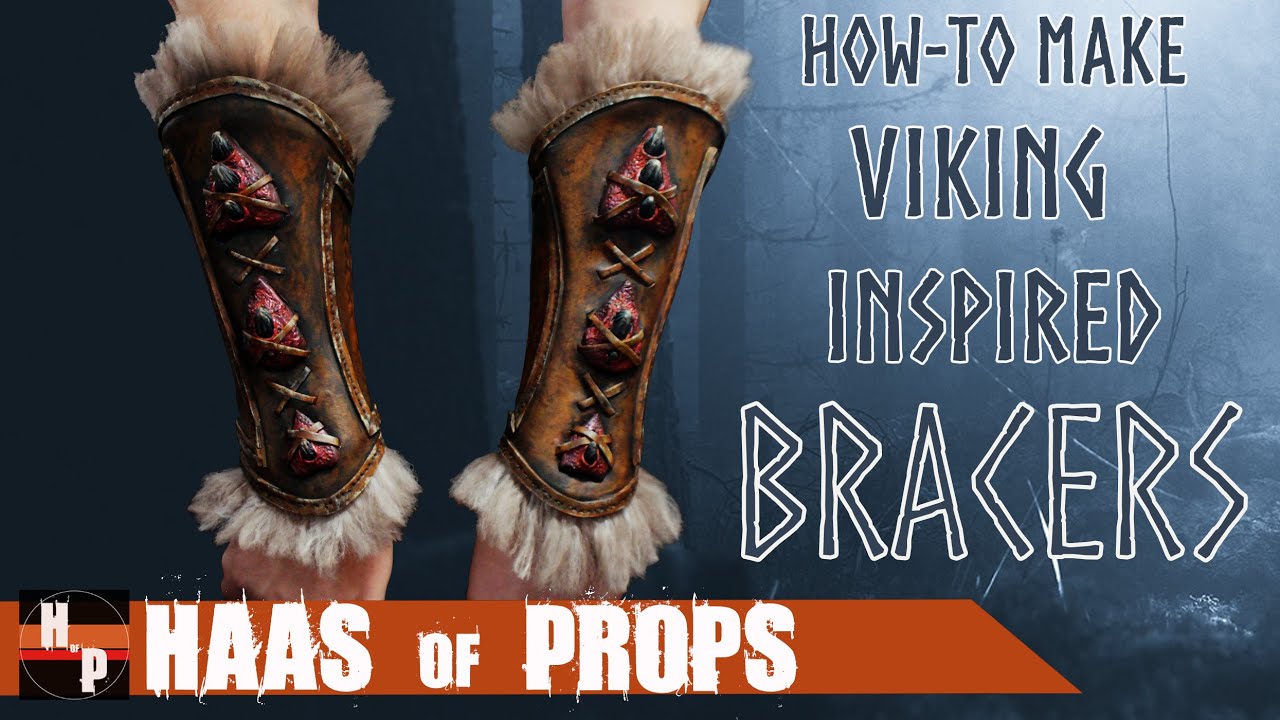A screen capture from a YouTube DIY video titled "How to Make Viking Inspired Bracers" is shown. The title is in all caps with stylized lettering on the right-hand side in a runic font. An orange banner at the bottom of the screen displays "HP, H-A-A-S House of Props" in white lettering, with an emblem in the bottom left corner. The bracers themselves are showcased on two arms, which could be either male or female, and feature fur-lined wrist and lower arm covers. They extend from the wrist to just below the elbow and exhibit decorations such as arrowheads or jewels and intricate leather ties with crisscross stitch patterns. The bracers are made from distressed brown leather with black and red accents, and white and cream fur peeking out at both ends. The background features varying shades of blue with a wintry, leafless wooded area to the right, enhancing the rugged, Viking aesthetic.